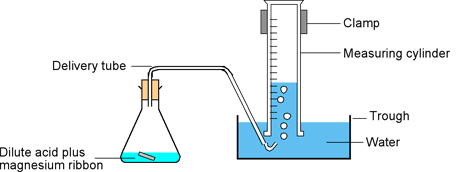The image is a detailed scientific diagram illustrating an experimental setup. On the left-hand side, there is a flask containing a bright blue liquid labeled as "dilute acid plus magnesium ribbon," with a small rectangular gray piece representing the magnesium ribbon. The flask is sealed at the top with a light brown cork, from which a delivery tube emerges. This tube extends upward at a 90-degree angle, turns, and then descends at a 45-degree angle into a larger container on the right.

The larger container, labeled as a trough, holds a dark blue liquid identified as water. White bubbles are seen rising from the end of the delivery tube submerged in the water, indicating a reaction occurring in the flask. The bubbles travel into a graduated measuring cylinder, also filled with water, positioned above the trough. The measuring cylinder is marked with black lines for measurement purposes.

Adjacent to the measuring cylinder, there are two clamps securing the apparatus. Various textual pointers label and describe each part of the setup, providing a clear understanding of the different components and their functions within the experiment.